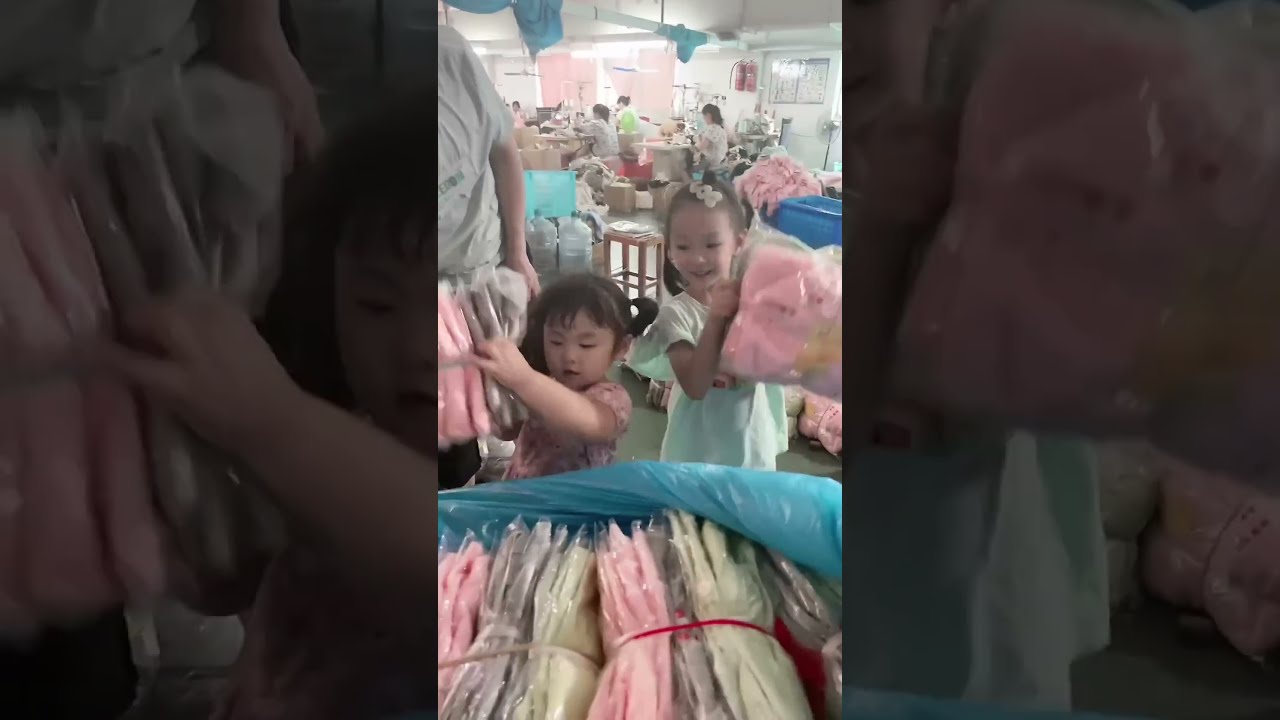In the center of this horizontally rectangular image, we see a young Asian man, slightly blurred, squatting down with his knees bent and sitting straight up. He wears a dark blue short-sleeved shirt, a Bluetooth earpiece in his right ear, and sports a decorative bracelet on his right wrist and a watch on his left wrist. His blue sneakers and a variety of fabrics, including pink and gray, are scattered around him. His arms rest on top of a heap of plastic packaging, likely containing clothing or other items, some of which are in a blue storage bin on the floor. The background shows a mess of boxes, books, and laundry baskets around a sunlit room with a window, adding to the disorganized scene captured in multiple slightly blurred close-up sections on either side of the main central image.